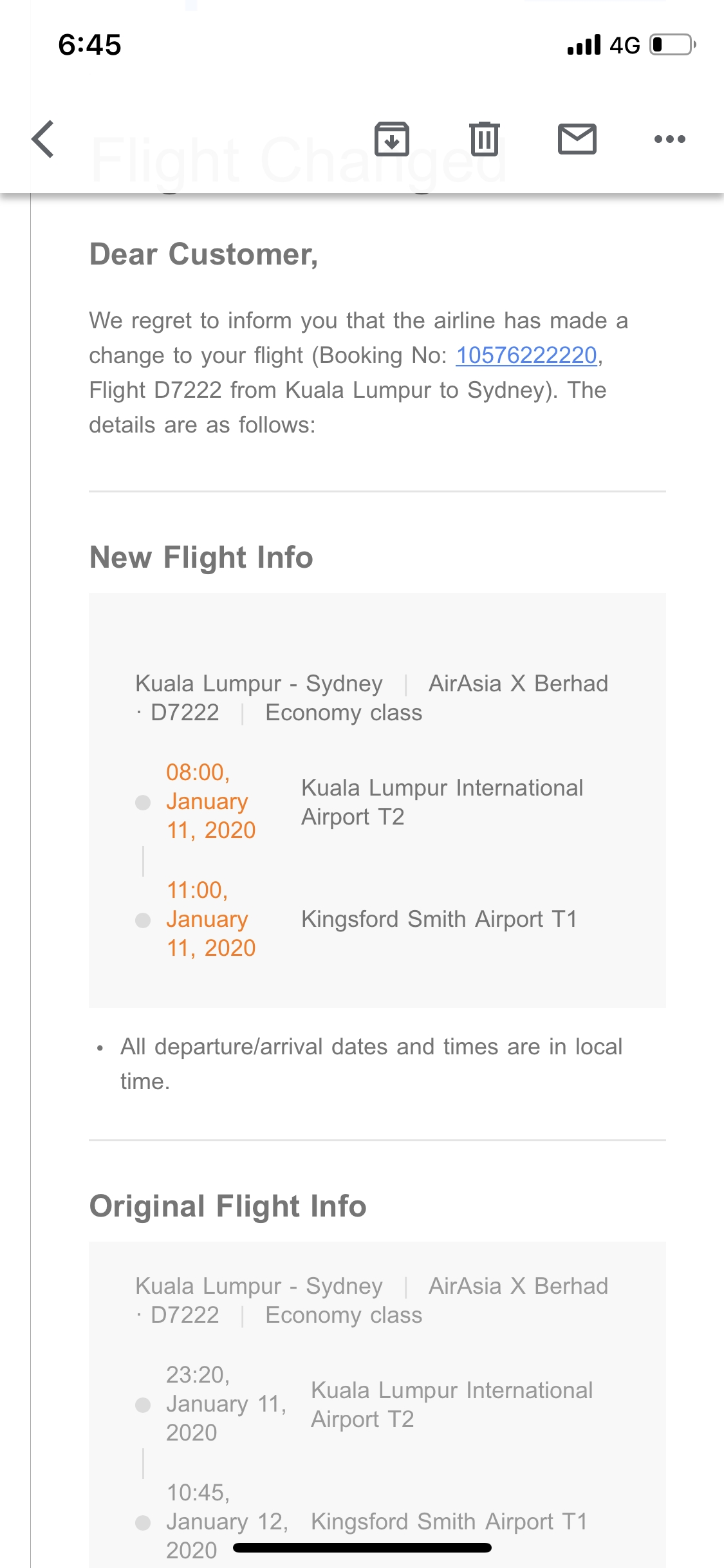Screenshot of a mobile device showing an email notification from an airline.

At the top of the device screen, the time displays as 6:45, with full signal strength indicated by four bars and a 4G connection. The battery level is around 20%. Icons at the top include a leftward-pointing gray arrow, a download arrow, a graphic, a trash icon, a mail icon, and three dots indicating additional options.

The email reads: 

"Dear Customer,

We regret to inform you that the airline has made a change to your flight. Booking number: [hyperlinked booking number]

Flight D7222 from Kuala Lumpur to Sydney.

Details are as follows:

**New flight information:**
- Kuala Lumpur to Sydney
- AirAsia, Flight D7222, Economy Class
- Departure: 08:00, January 11th, 2020, Kuala Lumpur International Airport, Terminal 2
- Arrival: 11:00, January 11th, 2020, Kingsford Smith Airport, Terminal 1

(All departure dates and times are in local time.)"

The original flight information is shown at the bottom of the email.